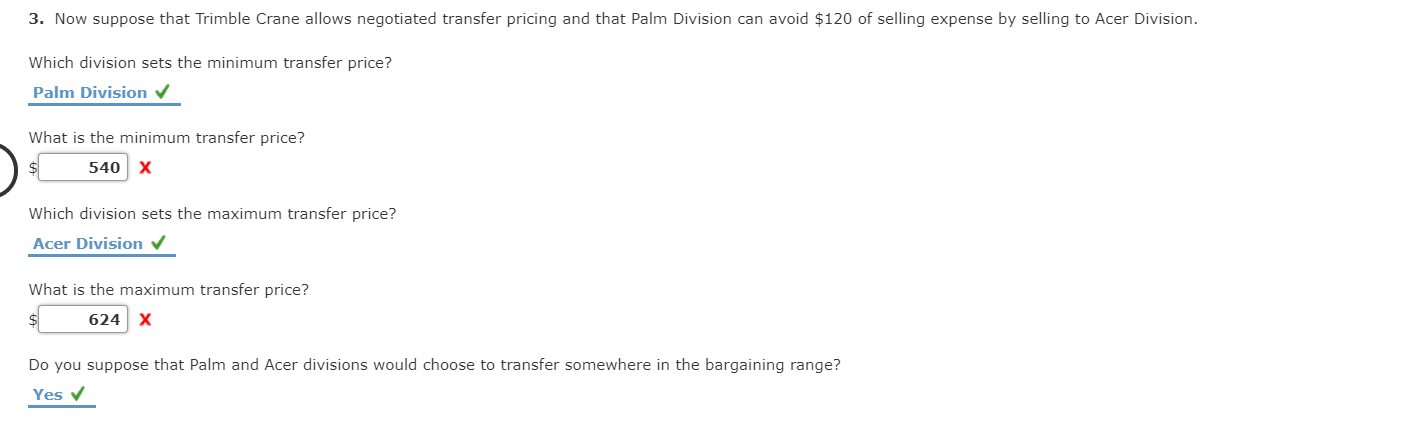This is a left-to-right horizontal image resembling a webpage view on a computer or smartphone screen with a white background. At the top, a partially visible sequence of numbers begins with the digit "3." Below, a statement regarding Trimble Crane's allowance for negotiated transfer pricing mentions that the Palm Division can save $120 in selling expenses by selling to the Acer Division.

Following this, a question asks, "Which division sets the minimum transfer price?" with the answer "Palm Division" displayed in blue and underlined, accompanied by a green checkmark. The next question, "What is the minimum transfer price?" is followed by a white box containing "$540," which has a red X next to it.

The text then inquires, "Which division sets the maximum transfer price?" The answer "Acer Division" is highlighted in blue and underlined, with a green checkmark beside it. For the question, "What is the maximum transfer price?" the provided answer "$624" appears in a white box, marked with a red X.

Lastly, the image poses the question, "Do you suppose that Palm and Acer Divisions would choose to transfer somewhere in the bargaining range?" The answer "Yes" is shown in blue and underlined, accompanied by a green checkmark.